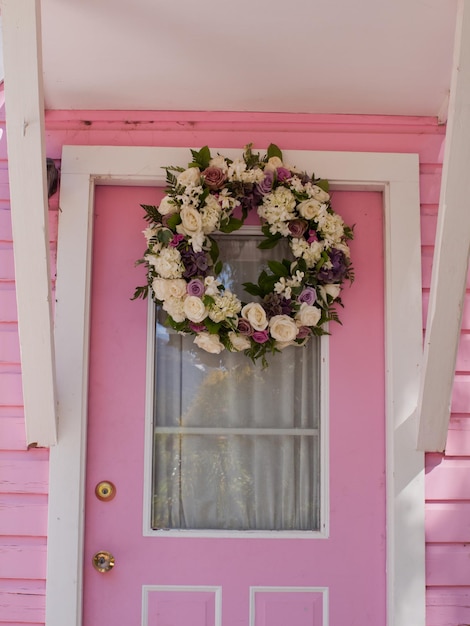This close-up photograph captures the entrance of a house painted in a striking bubblegum pink, featuring a door that matches the wall color. The door's trim is an off-white hue, and a small portico or awning, held up by diagonal beams, extends over the entryway, also painted in white. At the center of the door is a window, partially covered by an off-white curtain. The door's handle and lock are gold, positioned on the left-hand side. Adorning the top of the door is a large, round wreath composed of white and cream-colored flowers, as well as roses in shades of burgundy, pink, and rose, interwoven with greenery. The wreath's position partially overlaps the door frame, creating a charming, albeit slightly intrusive, decorative touch.